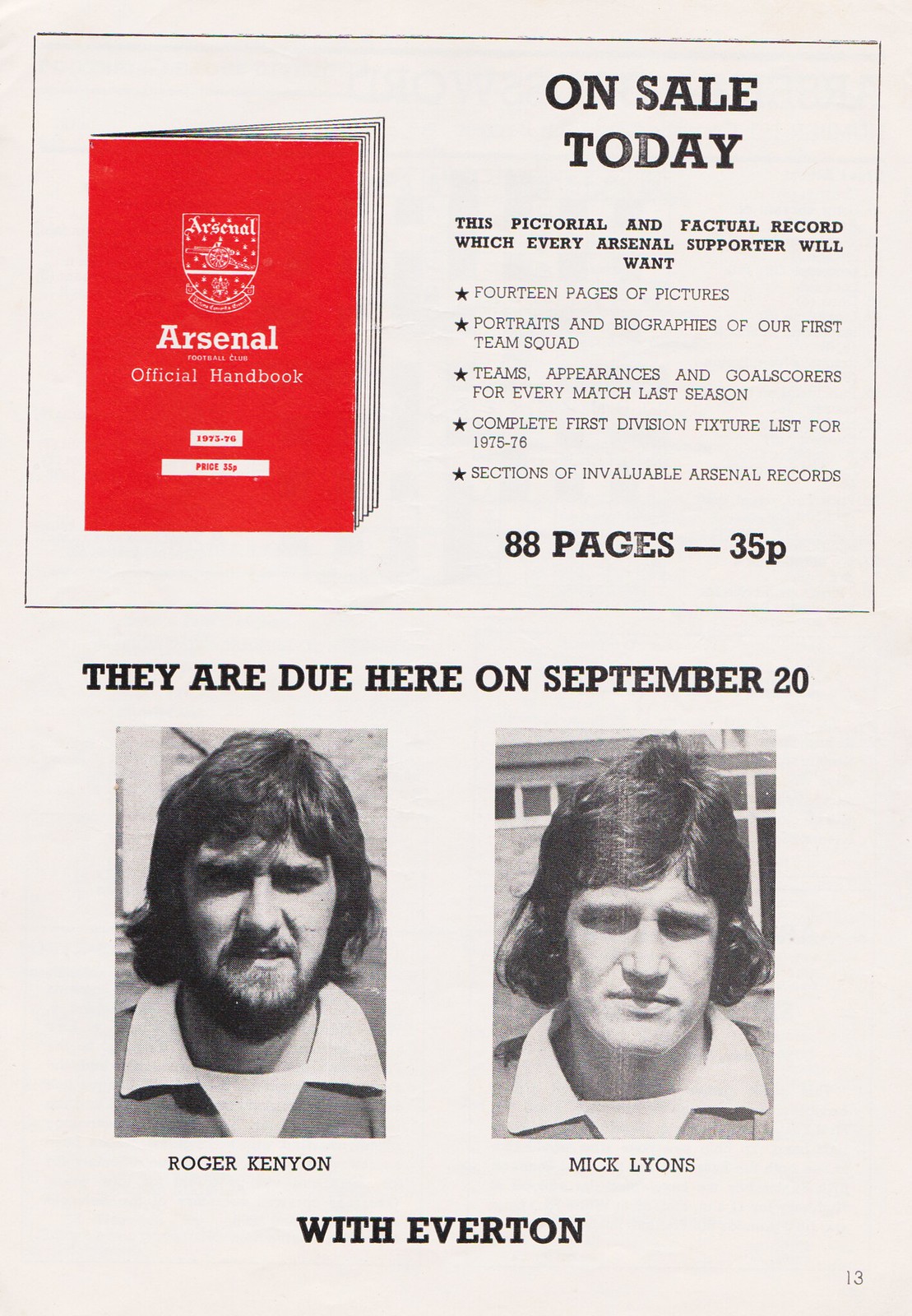The promotional flyer for the Arsenal Official Handbook features an off-white, light gray background with the number 13 printed in black in the bottom right corner, suggesting it could be part of a publication or a sequential flyer. The top half of the flyer is dominated by a white box framed with a thin black border. Inside this box, on the left side, is an image of a red booklet titled "Arsenal Official Handbook." To the right, black text promotes the handbook, highlighting its value to Arsenal supporters with detailed descriptions: "On sale today. This pictorial and factual record which every Arsenal supporter will want. 14 pages of pictures, portraits, and biographies of our first team squad, team's appearances, and goal scores for every match last season, complete first division fixture list for 1975 to 76, sections of invaluable Arsenal records." 

The bottom half of the flyer features black-and-white headshots of two individuals, identified as Roger Kenyon on the left and Mick Lyons on the right, accompanied by a caption stating they are due to appear with Everton on September 20th. The flyer as a whole measures 8.5 by 10 inches, and mentions the handbook has 88 pages priced at 35p.